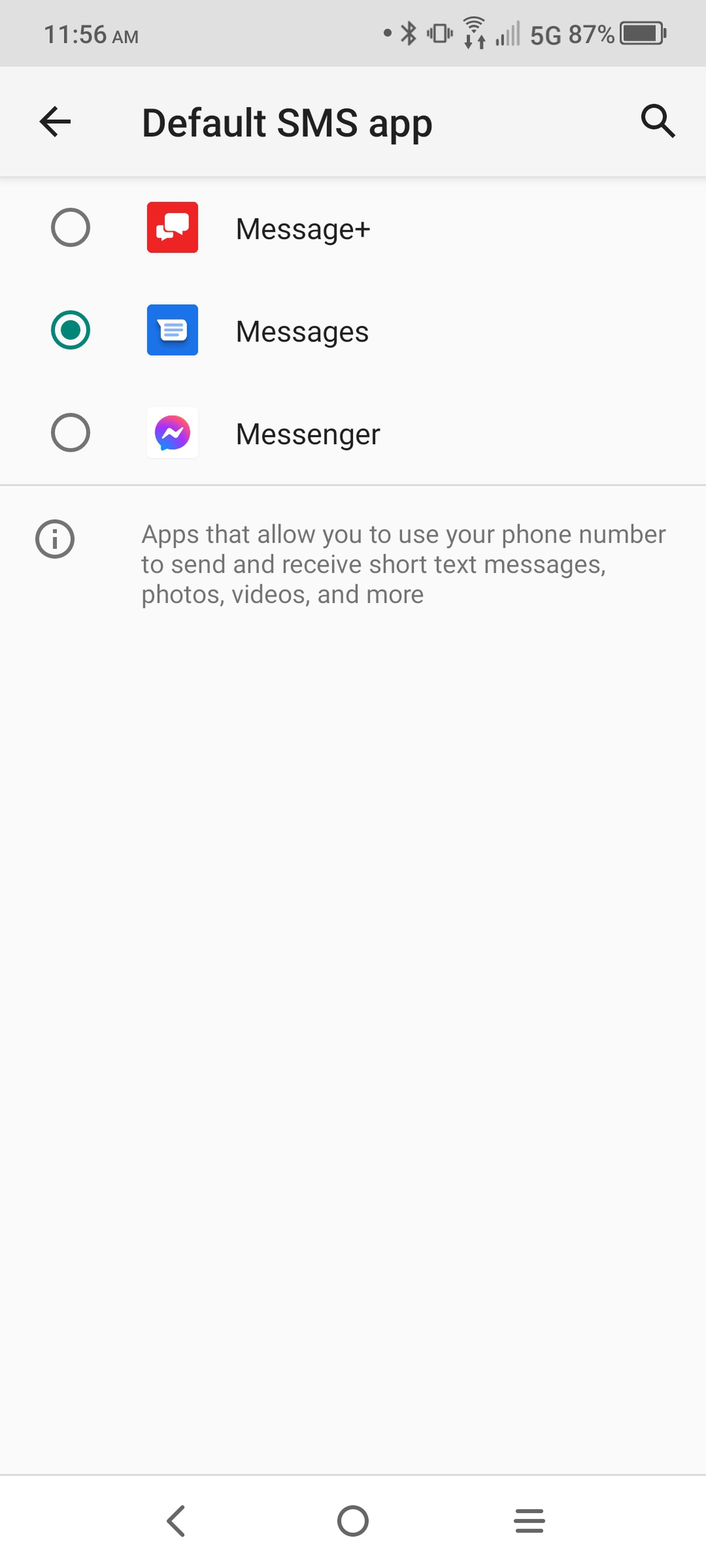A screenshot from a mobile phone displays at 11:56 AM, indicated at the top left corner. On the top right, icons for Bluetooth signal, phone sharing signal, WiFi signal, network signal, 5G connectivity, and battery percentage (87%) are present. The screen's background is light grey, while the header reads "Default SMS App" in black. Below this header are three options to select an SMS application:

1. **Message+** - Represented by a red icon with two white speech bubbles inside a square.
2. **Messages** - Depicted with a blue square icon containing a speech bubble with blue lines.
3. **Messenger** - Shown with a colorful gradient background (blue, purple, and red) and a speech bubble with a stylized white 'N' inside.

Beneath these options, grey text next to an eye symbol explains, "Apps that allow you to use your phone number to send and receive short text messages, photos, videos, and more."